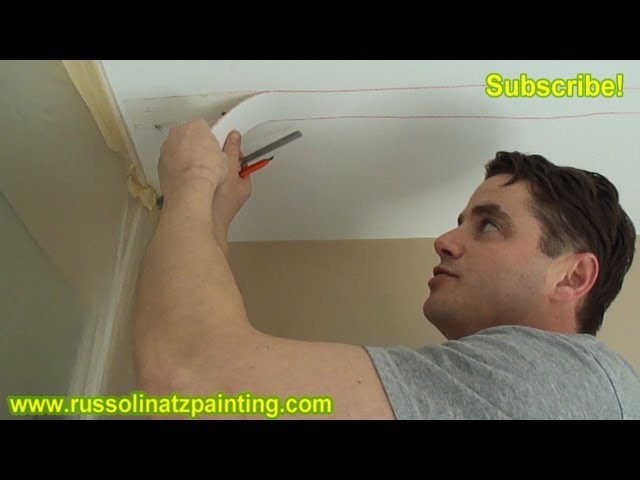In this rectangular, letterboxed photograph, a Caucasian man in a gray t-shirt is seen meticulously working on a white ceiling from an elevated platform, possibly a ladder. The man, who has short, wavy brown hair, is engaged in peeling off a strip from the ceiling, which he had previously marked with red lines using a marker. He also appears to be holding a ruler and a fine red tool, likely a knife or pen. The man is positioned against beige walls on the left and right side of the image. In the top right corner, yellow text reads "Subscribe!" and in the bottom left corner, the website "www.russellenutspainting.com" is displayed.